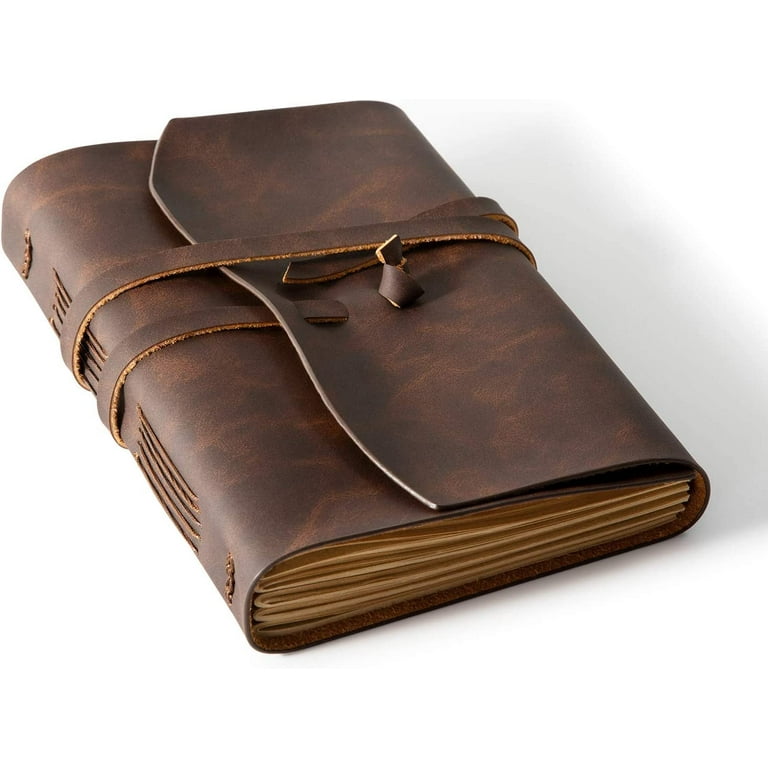The image is a photograph of a dark brown, leather-bound book or journal, possibly handmade, set on a plain white surface with a slight shadow to the right. The rich leather cover features a strap that wraps around the book to keep it securely closed, with the strap tied in a knot. The texture of the leather is detailed, with some shading and mottling giving it an old-fashioned, almost rustic look. The front cover extends over the spine and halfway to the back, where decorative slits run in two columns along the spine, each column possessing several evenly spaced slits reminiscent of Old West styling. Inside, the book contains slightly yellowed pages that appear to be loosely bound, indicative of handmade binding or folded and stapled pages. There are also hints of lighter paper or possible manila envelopes visible from the bottom. Overall, the book's ornate yet simplistic design suggests it could be a journal, a Bible, or an old ledger, potentially emphasizing its vintage and craftsman-like allure.